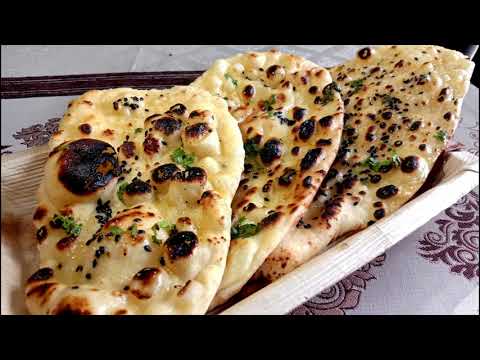The wide rectangular photograph features a dish of Indian naan bread elegantly placed inside a beige, rectangular cardboard-looking plate positioned on a white fabric surface adorned with embroidered maroon floral patterns, visible in the bottom right, top left, and slightly on the top right corners. The three naans, somewhat oval in shape, rest atop one another within the plate. These naans display large burnt spots of varying sizes, adding a rustic touch to their very light cream, almost whitish-yellow, puffy texture. Scattered across the naans are white dots as well as sprinkles of green parsley, enhancing their visual appeal. The entire ensemble sits atop a white tablecloth subtly decorated with curling lines and floral designs, contributing to the image's detailed and textured composition.